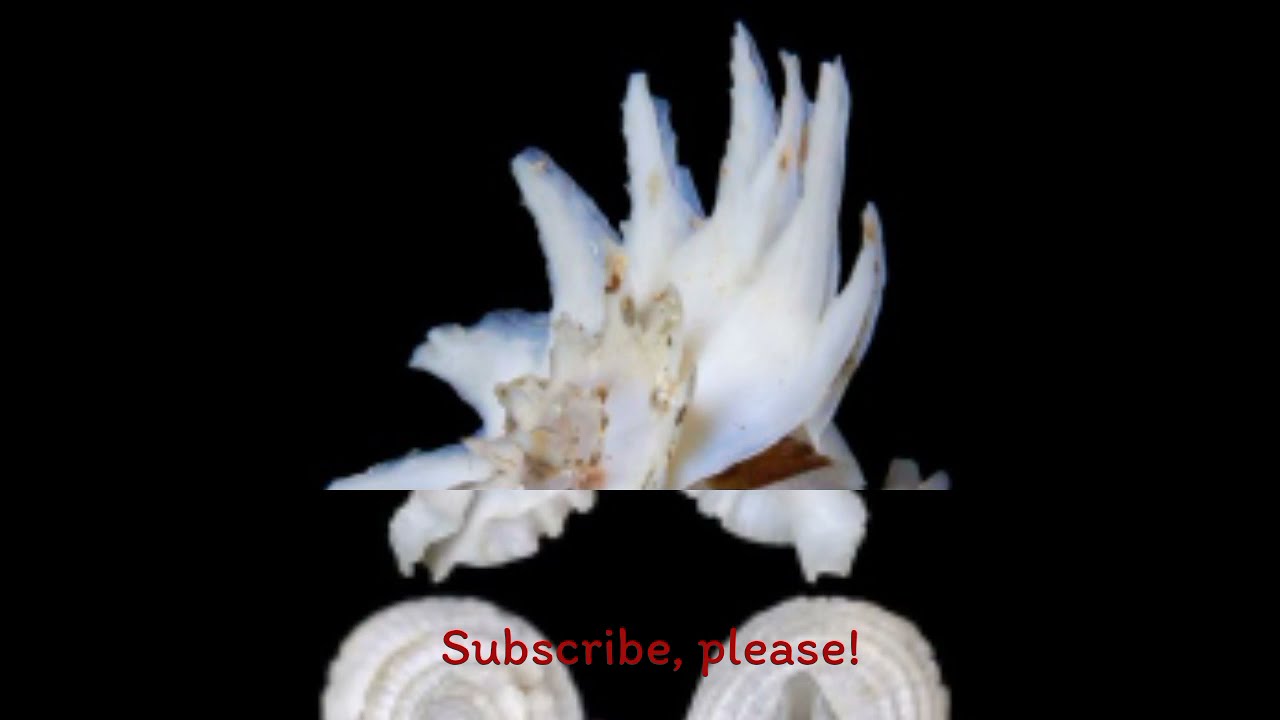The image has a black background and appears somewhat disjointed, possibly the result of two separate images combined. At the center is an ambiguous white object with multiple points, resembling either petals of a flower, starfish, or a seashell, characterized by light blue, beige, tan, and brown markings. This object somewhat mimics the form of dove wings beneath it. The bottom portion of the image features red text reading "subscribe please!" topped off with an exclamation mark, and two white circular objects resembling onion slices, showing their concentric rings. The image is a horizontal rectangle, likely designed for use on a social media account or a website.